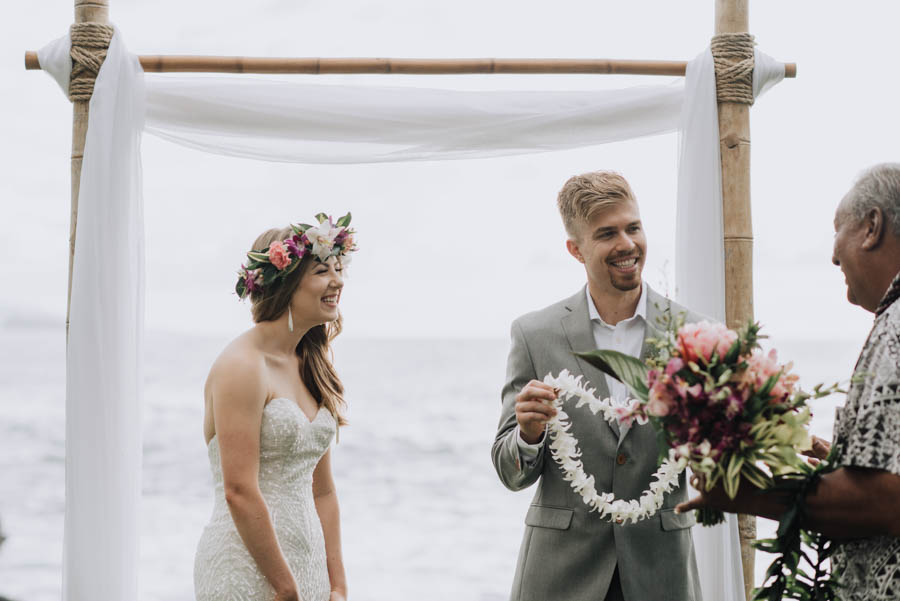In this beachside wedding, a young white couple stands beneath a bamboo arch adorned with white lace wrapping. The bride, dressed in a strapless white evening gown and pearl drop earrings, has a flower crown nestled in her long brown hair. She holds a bouquet of flowers. The groom, in a gray suit with a white shirt, sports blonde hair and a mustache-goatee combination, and he holds a white flowered lei. The officiant, likely an islander with darker skin, wears a tropical-style black-and-white shirt and holds a bouquet of pink peonies with greenery. They are positioned in the center of the horizontal photo, with the ocean visible behind them, reflecting the cloudy, overcast sky.